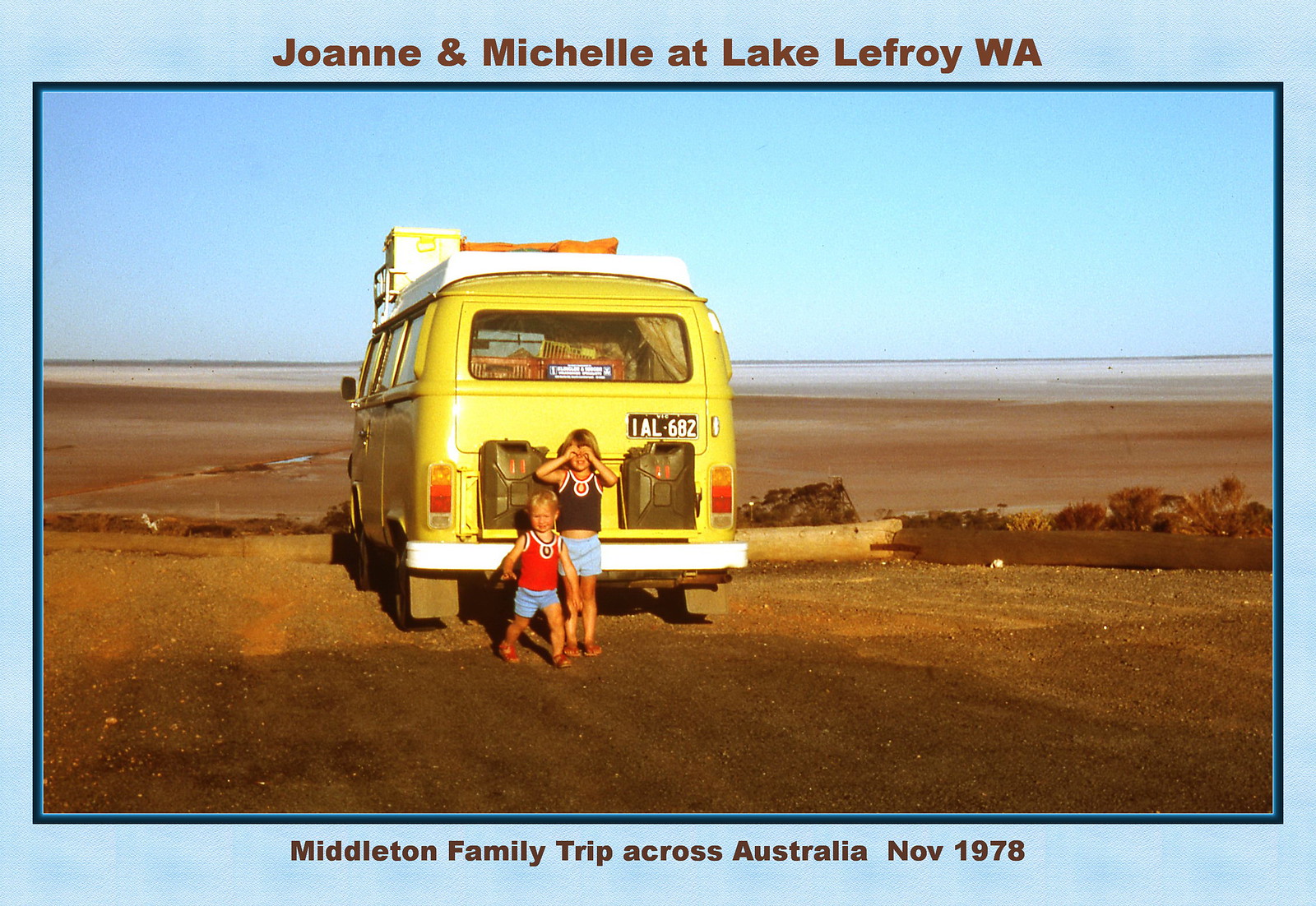This vintage postcard depicts a yellow Volkswagen bus parked in a gravel lot at Lake Lafroy, Washington, against a backdrop of clear blue skies and a sandy beach leading to the sea. The bus, packed for travel with suitcases and baskets visible through the rear window, features two young children standing at the back, likely around two and four years old. One child is shielding their eyes from the sun, dressed in summer clothing including shorts, tank tops, and sandals. Above the photo, framed by a light blue border, the inscription reads "Joanne and Michelle at Lake Lafroy, Washington" and below the image, it says "Middleton family trip across Australia, November 1978."